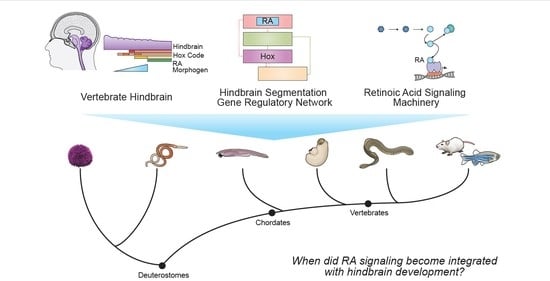This image is a detailed scientific diagram focused on the evolution of the vertebrate hindbrain and the integration of retinoic acid (RA) signaling in its development. In the upper left corner, there is a cutout diagram of the human brain, labeling the hindbrain, the Hox code, and RA morphogen. The top middle section presents these elements stacked in rectangular images as part of a hindbrain segmentation gene regulatory network, while the upper right corner depicts elements being sequenced and is labeled as retinoic acid signaling machinery. An evolutionary flowchart, faintly marked by blue arrows pointing downwards, runs beneath these sections. This flowchart is labeled "deuterostomes," "chordates," and "vertebrates," respectively, and includes visual examples such as a worm, a snake, rats, and fish, illustrating the progression of how animals evolved up to vertebrates. The diagram as a whole seems to be attempting to elucidate when RA signaling became integrated with hindbrain development within the evolutionary timeline.